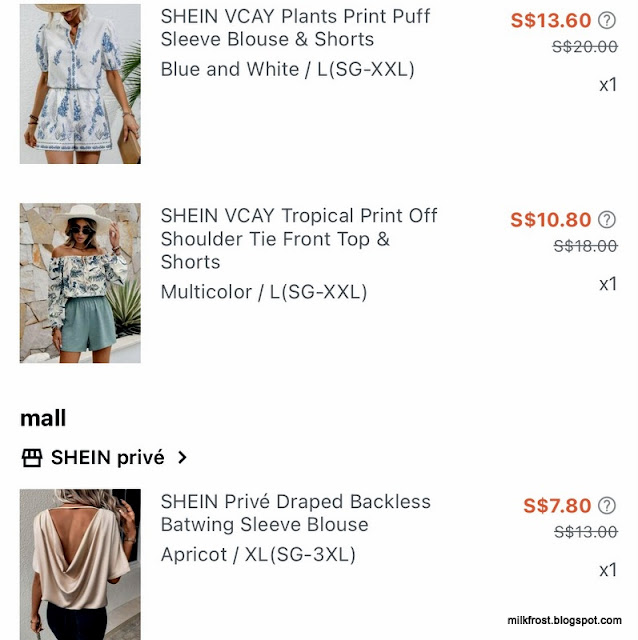This is a detailed caption for an online shopping website, specifically Shine, which offers a variety of affordable clothing and items:

---

The screen displays a portion of Shine's website, known for its budget-friendly online clothing and accessories. The top of the page prominently features the brand name "SHINE" in bold, black capital letters against a clean white background. Just below this title, the product listings commence.

### Product 1: 
**VCAY V-K Plant Print Puff Sleeve Blouse and Shorts Set:**

- **Description**: This set includes a white blouse with blue plant prints, featuring puff sleeves, and matching shorts.
- **Size Range**: Available from Small (S) to 2X-Large (2XXL).
- **Price**: Originally listed at $20, now marked down to $13.60.
- **Image**: Displays the blouse and shorts, highlighting the plant print design.

### Product 2: 
**VCAY Tropical Print Off-Shoulder Tie Front Top and Shorts Set:**

- **Description**: A colorful, off-shoulder top with a tie front, paired with matching shorts featuring a tropical print.
- **Size Range**: Available from Small (S) to 2X-Large (2XXL).
- **Price**: Originally $18, now reduced to $10.80.
- **Image**: Shows the vibrant top and shorts set.

### Product 3:
**Privet Draped Backless Batwing Sleeve Blouse:**

- **Description**: An apricot-colored blouse with draped back and batwing sleeves.
- **Size Range**: Available from Small (S) to 3X-Large (3XXL).
- **Price**: Originally $13, now discounted to $7.80.
- **Image**: Displays the apricot blouse with its unique draped back design.

On the left side of the screen, there is also a navigation label "MALL" underlined by a small black storefront icon. Below this, it reads "SHINE PRIVE" with an arrow pointing right.

### Footer:
At the bottom right, a watermark indicates the source of the image as: "milkfrost.blogspot.com."

---

This comprehensive caption provides a clear and detailed description of the Shine website's content, highlighting specific products, their designs, prices, and available sizes.